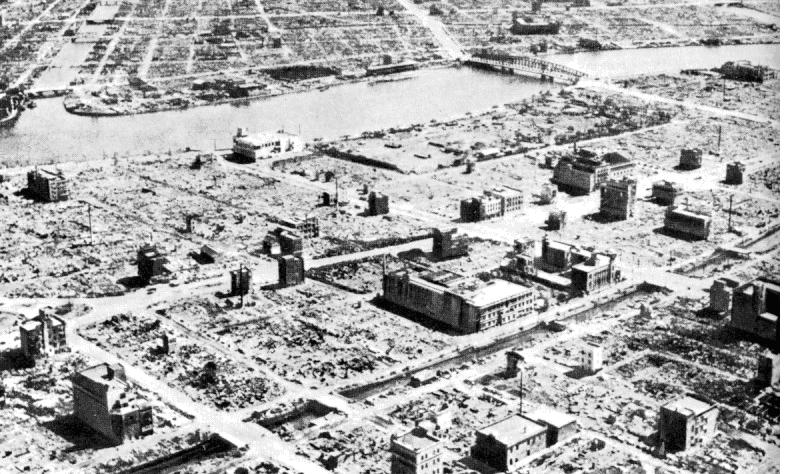This black-and-white photograph captures a devastated cityscape, possibly after a major storm or other form of destruction. The image showcases a city laid out in a grid pattern, with plots of land where buildings once stood, now largely empty or reduced to rubble. Only a few scattered, multi-story buildings remain, ranging from four to six stories tall, accentuating the sparsity and widespread devastation. The streets run at right angles, orderly despite the chaos, and some land areas appear to be just dirt, indicating where structures might have been completely removed or washed away. 

In the background, a large river runs horizontally with a bridge crossing it, and the city extends beyond the river, following the same pattern of destruction. Some of the buildings are perilously close to the water’s edge, hinting at possible flooding. The lack of dense construction and the visible damages strongly suggest that this city is either in the early stages of rebuilding or is a sobering post-storm landscape. The absence of color enhances the somber tone and highlights the severity of the destruction seen in this historic photograph.